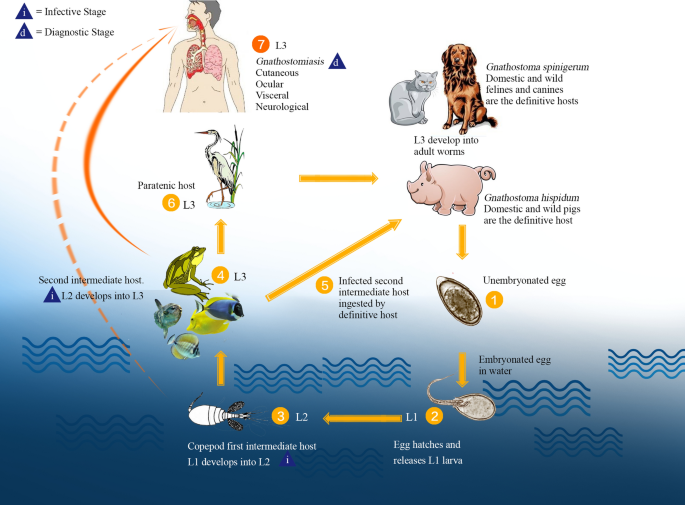This detailed diagram illustrates the transmission pathways and effects of a parasitic infection affecting both humans and animals. In the top-left corner, it highlights the infective and diagnostic stages with a picture of a human showing lung issues. The primary labels include "ocular," "visceral," and "neurological," indicating the affected organs and symptoms. The human host is infected by a complex chain extending through several intermediate hosts: copepods, frogs, fish, and birds. This infection cycle branches out to show that dogs, cats, and pigs are also involved. Dogs and cats, both domestic and wild, can host and develop the worms, while pigs serve as another intermediate link, passing unembryonated eggs into water sources. The chart uses distinct colors—orange, blue, green, gray, pink, and brown—to differentiate various elements and stages, with a blue squiggle pattern covering the lower half of the diagram, enhancing visual segmentation.